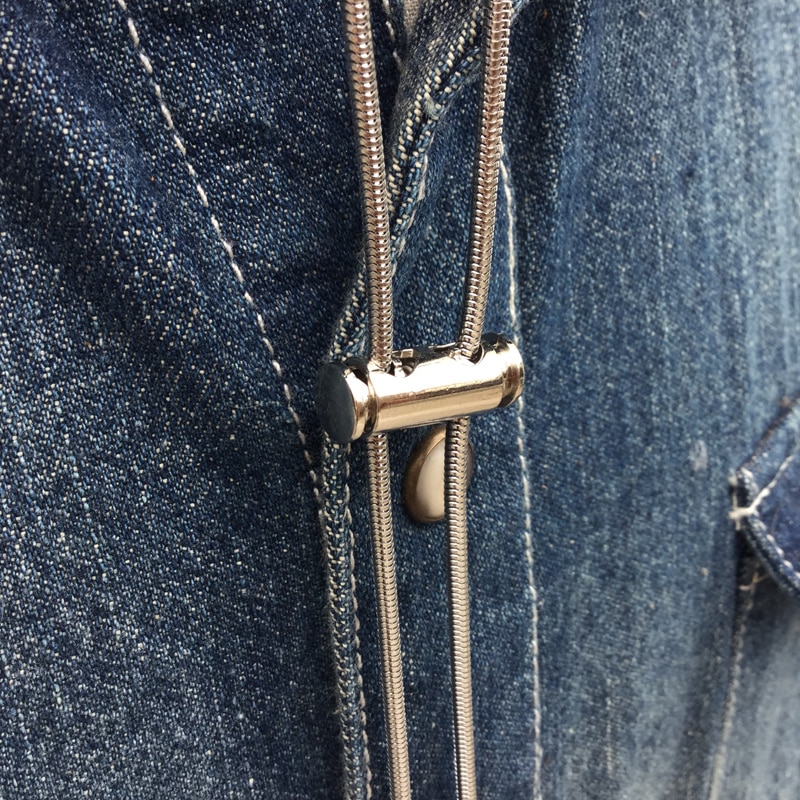The photograph is a close-up image of a gold-colored metal rope accessory, resembling a bolo tie or detailed drawstring, set against a backdrop of dark denim fabric. This denim fabric features prominent white stitching, and a portion of a pocket is visible in the bottom right-hand corner. The metal rope appears coiled and is joined by a shiny gold cylindrical piece with holes, enhancing its decorative and possibly functional design. This cylinder and rope ensemble sits near what looks like a button, suggesting that the background garment is likely a jacket, contributing to its overall look as a Western-style accessory. The image captures the intricate detailing of both the rope and the denim, highlighting the contrast between the metallic accessory and the textured fabric.